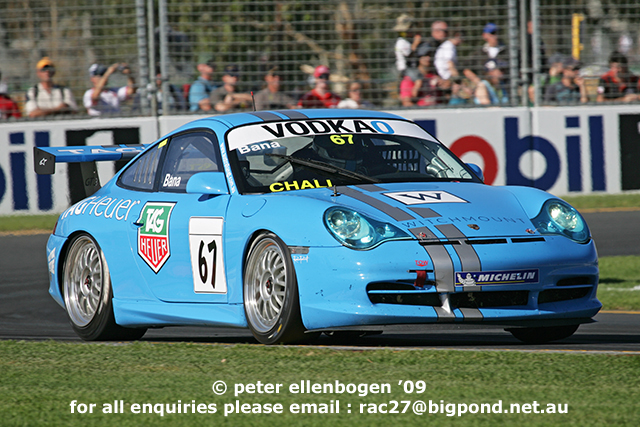The image captures a vivid racing scene set outdoors in the middle of the day on a well-worn asphalt track. The track is bordered with patches of low-cut grass, and towards the top of the image, a wall and a fence contain a crowd of spectators, including several fans eagerly watching the action. Prominent billboards with various brand names can be seen behind the fence.

At the heart of the photograph is a striking light blue race car, positioned centrally in the frame. The car, identified as number 67, features multiple advertisements. The driver's side door sports a white square with the number 67 in black text. Visible branding includes "VODKA" or possibly "ROCKO," and other labels such as "TAG HEUER" on the side, "MICHELIN" on the front, and something like "WITCHMOUNT" on the hood, accentuated with gray racing stripes.

The car's dynamic stance shows it pointing towards the lower right corner from the front, with its back end angled towards the left middle of the image. Additional text and logos appear on the windshield: "BANA" on the right corner, "67" in the middle, and "CHALI" on the lower right part.

Underneath the main caption, a copyright notice reads, "Peter Allenbogen 09. For all inquiries please email rec27 at bigpond.net.au." The colors in the image are varied, with green grass, the gray asphalt, light blue and white on the car, and accents of red and yellow.